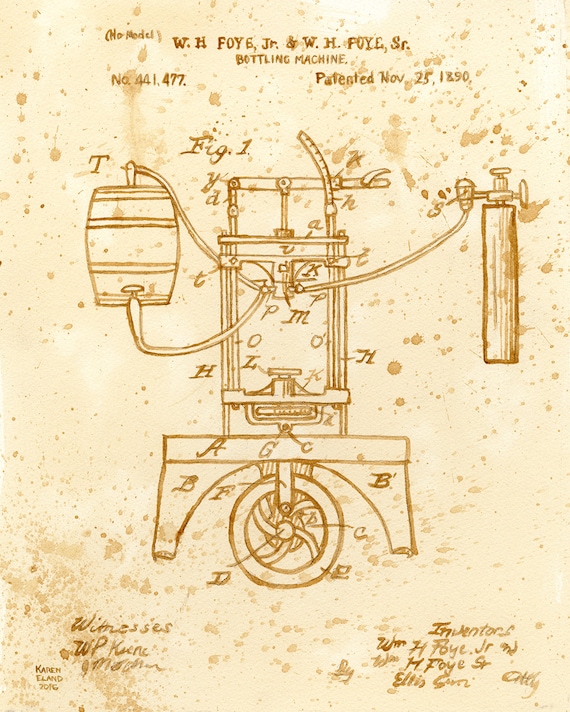This image is an intricate, antique pen and ink sketch on yellowed paper, showcasing a detailed schematic for a bottling machine patented on November 25, 1890. The drawing, possibly executed with a quill in brown ink on a beige background, features a complex array of mechanical components including a wheel at the bottom, interconnected hoses, and various gears and pumps. At the top, the names "WH4Jr", "WH4Sr", and the Model "WH Foy" are inscribed, indicating the inventors. Key details like "Witnesses" and "Inventors" are positioned in each corner at the bottom of the page. Despite being sprinkled with stains and showing signs of age and damage, the sketch appears authentic, though a small inscription "Karen Eland, 2016" in the bottom left suggests it might be an artistic drawing rather than an original schematic.